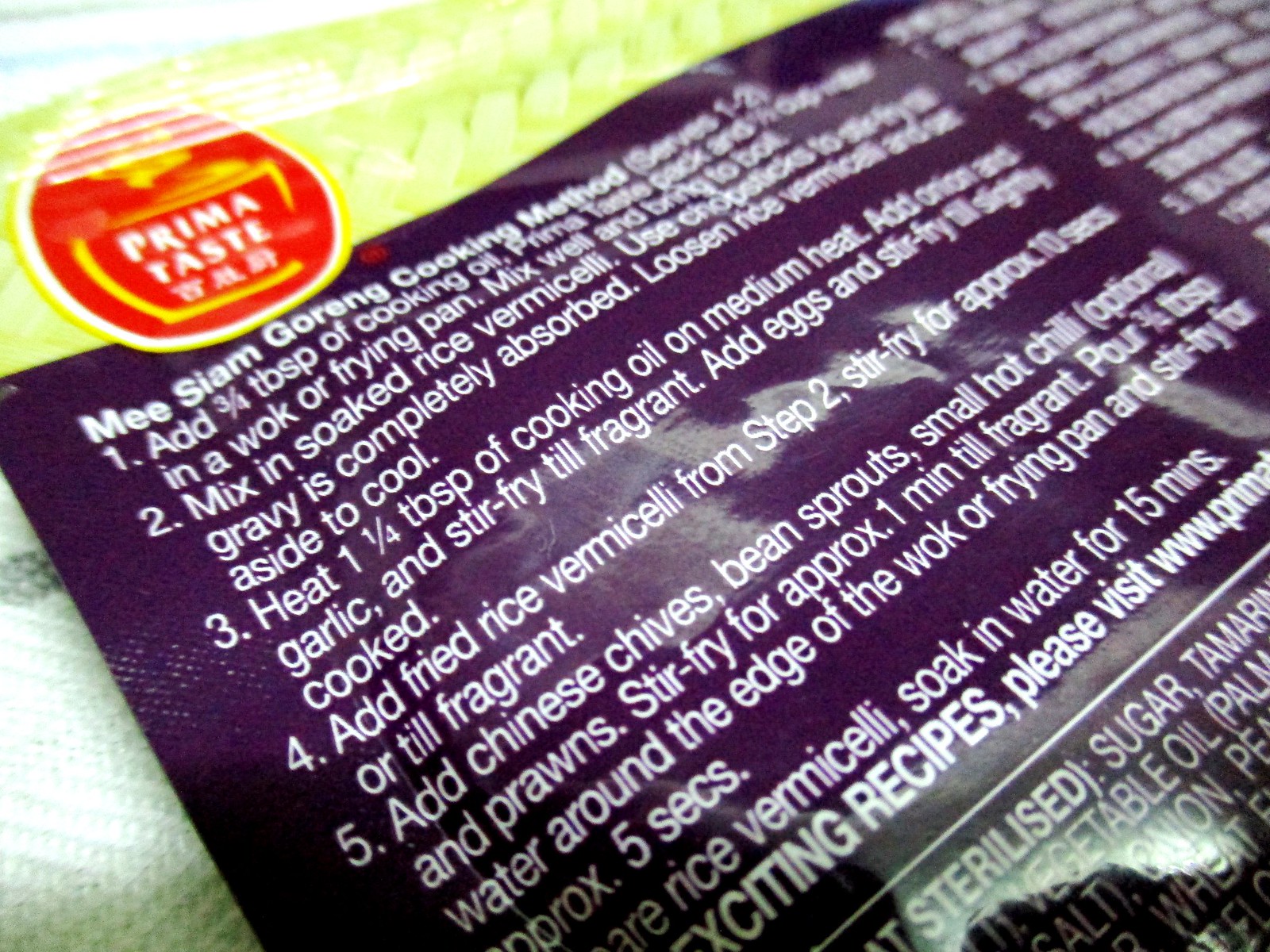The image shows the back of a Prima Taste food package, likely for rice vermicelli Mi Siam Goreng, featuring detailed cooking instructions and partial ingredients. The logo, positioned at the top left, consists of a red circle with "Prima Taste" in white and three Asian characters below it. The logo also includes a yellow outline of a bowl with steam. The background is primarily purple and displays the Mi Siam Goreng cooking method intended to serve one to two people, broken down into detailed steps. Instructions include adding and heating cooking oil, stir-frying onion and garlic until fragrant, adding eggs, incorporating soaked rice vermicelli, and mixing in optional ingredients like chives, bean sprouts, and prawns. The last step involves pouring water around the edge of the pan. The bottom section, mostly cropped out, lists partial ingredients such as sugar, vegetable oil, onions, wheat, tamarind, and palm oil. Overall, the focus is on the five-step cooking method highlighted against the purple backdrop.